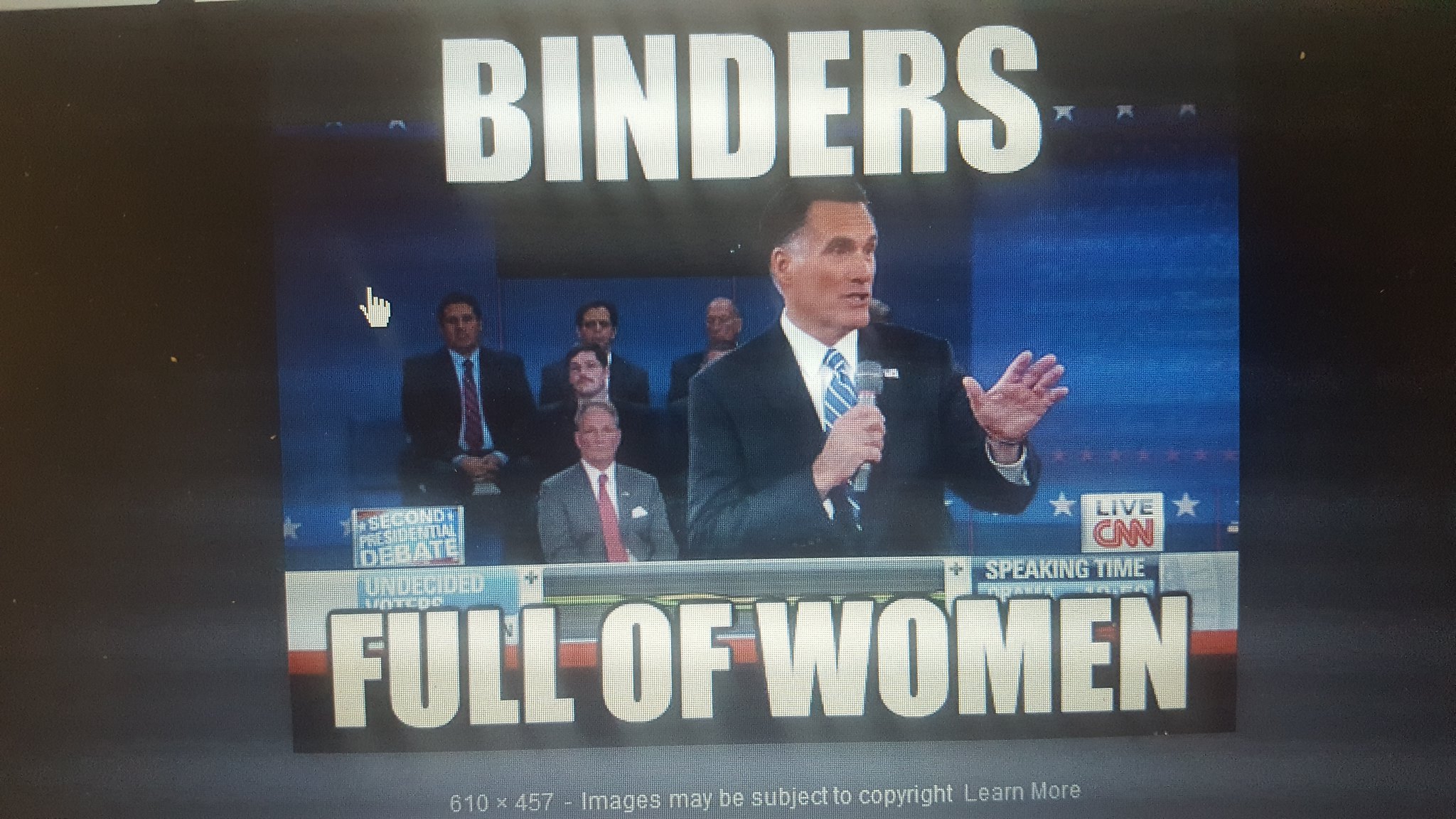This is a screen capture taken from a live CNN broadcast of a U.S. presidential debate, depicting Representative Mitt Romney mid-speech. Positioned at the center, Romney is shown holding a microphone in his right hand, while his left hand is raised, palm visible. He is slightly turned to his left, dressed in a dark suit, blue tie with white stripes, and a white shirt. His hair is dark with distinctive white sideburns. 

In the background, there are six men who appear to be seated on a panel or riser, attentively listening to Romney. The image has the feel of a meme, with overlaid white, capital letters at the top reading "BINDERS" and at the bottom "FULL OF WOMEN," referencing a notable phrase from Romney during the debate. The screen has the "live CNN" logo and additional text indicating "second presidential debate, undecided voters," though some of the text is unreadable.

The overall captured image is set against a dark gradient background, lightening towards the bottom, where white text reads "610 by 457 - Images may be subject to copyright. Learn more," suggesting this is a screen capture from a video or digital format. The sides of the image are bordered in black, completing the layout typical of a meme-style presentation.